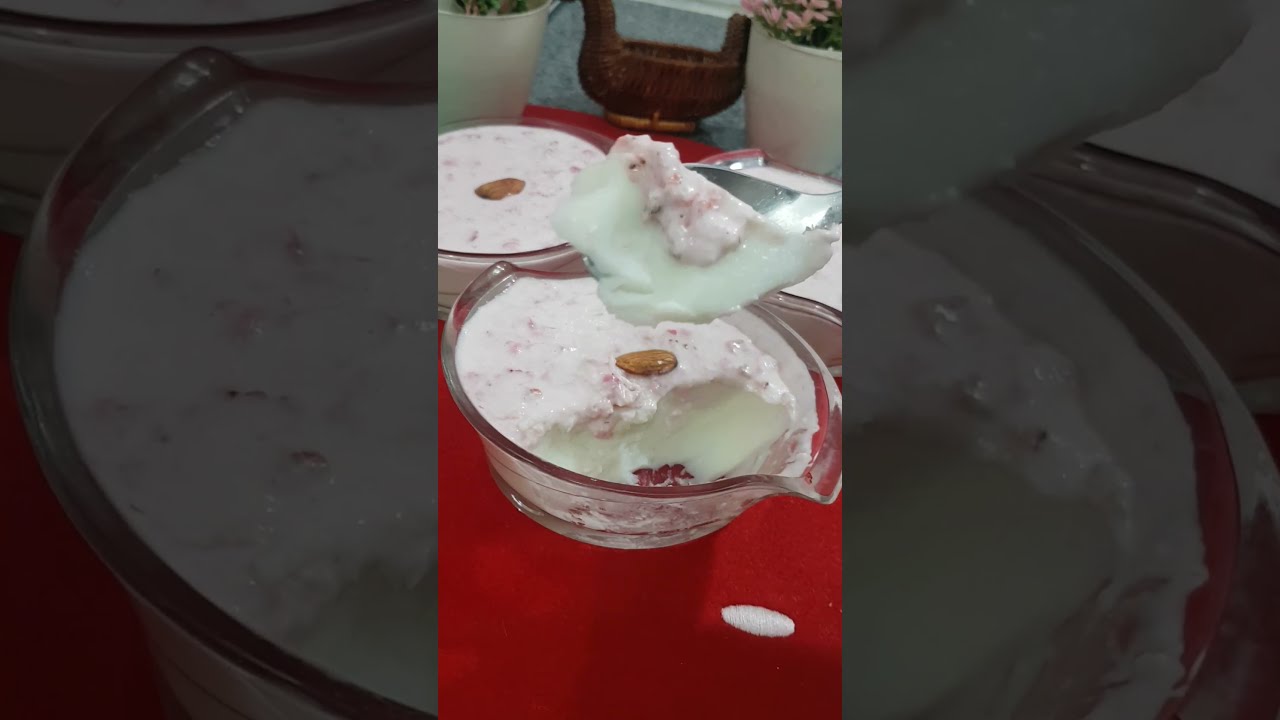The image captures a zoomed-in scene of someone watching a YouTube video on their phone. Centrally framed within the up-close shot is another photograph showcasing a delectable dessert presented in glass dishes. Each dish holds a smooth, white pudding topped with a layer of creamy, strawberry-like substance and an almond nestled at the center. The main focus is on a spoon lifting a portion of the dessert from one of the dishes, with a small droplet having fallen onto the bright red surface below. In the backdrop, there’s a second identical dessert, slightly to the left. This setting is further accentuated by two white pots featuring light pink flowers and an ornate wooden animal basket positioned between them, all resting on a red table, possibly covered with a tablecloth. The side portions of the image are framed with gray, presumably due to the phone's interface displayed in the screenshot.